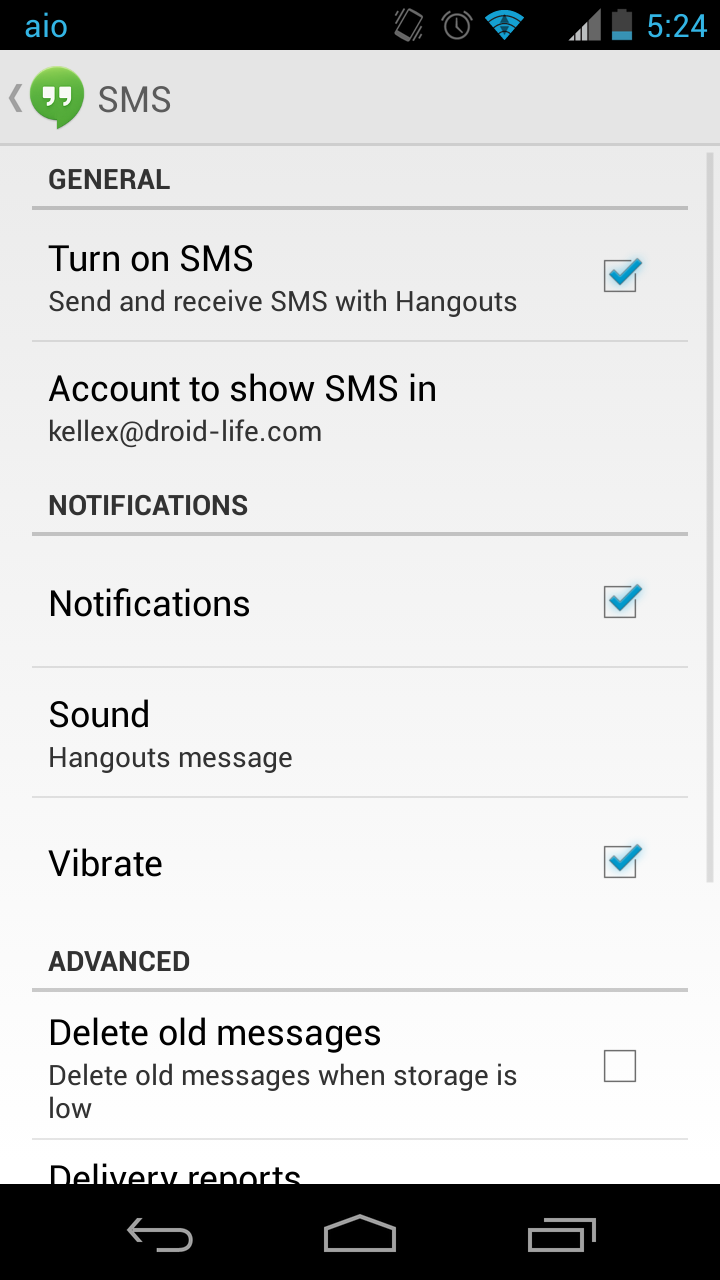Screenshot of an Android phone displaying the SMS settings menu. At the top, under the "General" category, there's an option to "Turn on SMS" which is enabled, indicated by a blue check mark in a square. Below it, "Account to show SMS" displays an associated email address. Moving down, the "Notifications" section includes a sound setting labeled "Hangouts message" and a vibrate option. The "Advanced" section features an option to "Delete all messages," and a setting for "Delivery reports." Each section is visually separated by gray lines against a gray background, with all text in bold black. The interface ends with the standard Android navigation buttons: back, home, and multitask, located at the bottom of the screen.